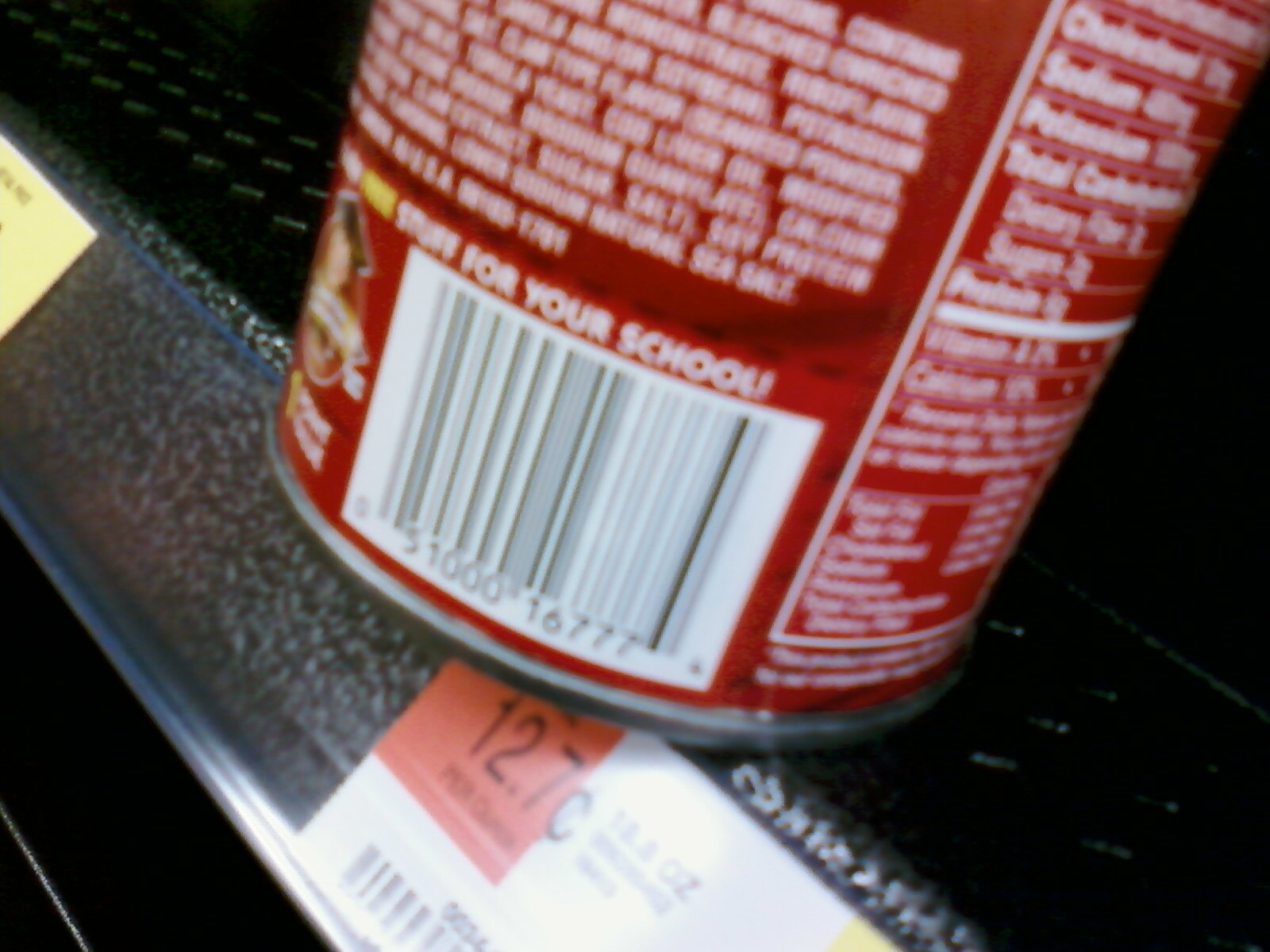This close-up image features the bottom portion of a Campbell's Soup can sitting on a black, shiny, metal store shelf. The can, wrapped in its iconic red label with white writing, prominently displays various details, including a QR code and nutrition information along the curved side. On the bottom right-hand curve, the Campbell's Soup mascot is visible. The can also has "Win free stuff for your school!" and a partial barcode. The shelf, angled diagonally from the bottom right to top left corner of the image, has a white and orange price sticker labeled 12.7C, although some of the sticker's information is obstructed. The image also captures part of the ingredients list and nutritional details, though they are blurry and difficult to read.